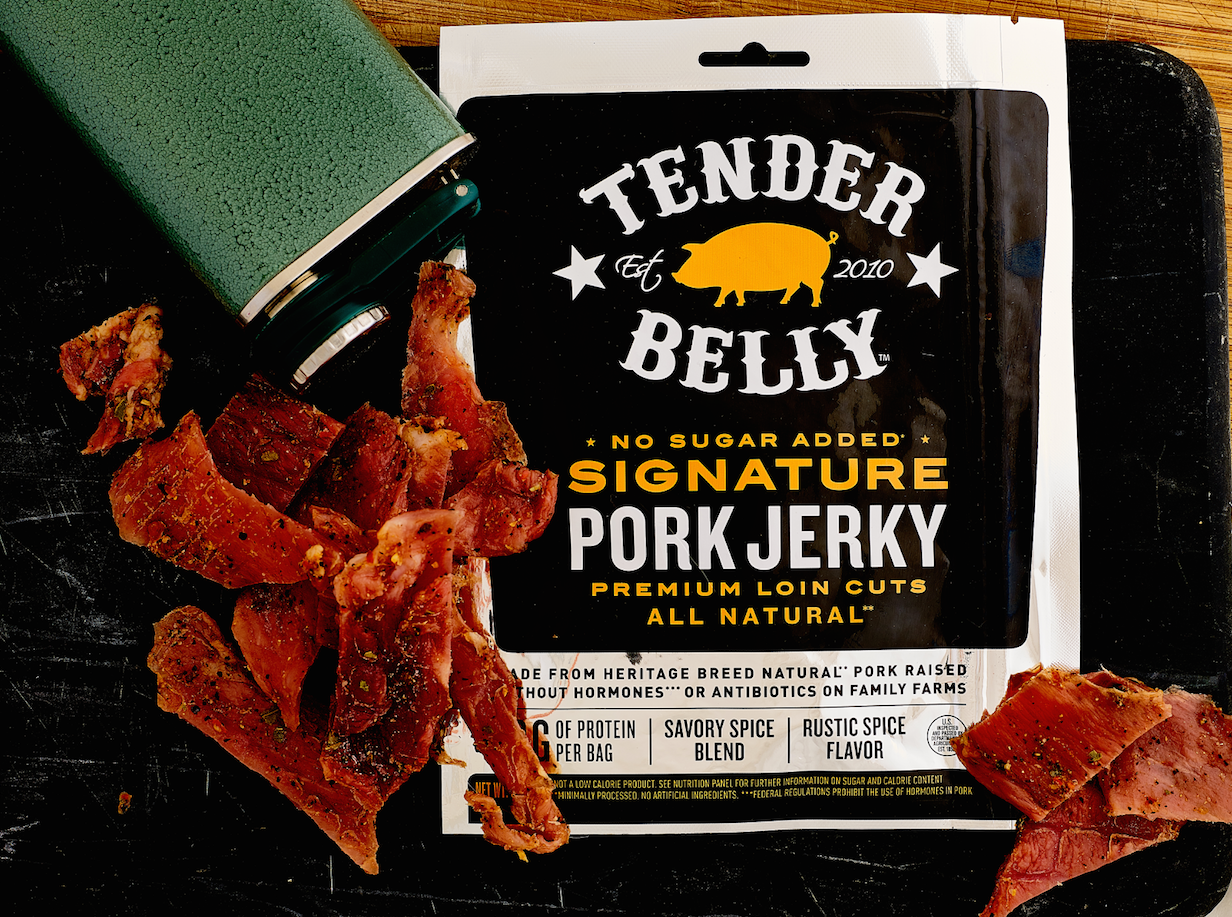The image showcases a vividly colored package of pork jerky under the brand "Tender Belly," clearly labeled in bold, white, all-caps letters. The logo features a small pig, colored yellow, next to the text "Established 2010." The packaging prominently states "No Sugar Added," "Signature Pork Jerky," "Premium Loin Cuts," and "All Natural," along with additional details that the pork is made from heritage breed, natural pork raised without hormones or antibiotics on family farms. The design suggests a natural and wholesome product with a rustic spice flavor. Spread across the black pad beneath the packaging, there is a large, seasoned pile of light red pork jerky on the left side, with some pieces also scattered on the lower right. The jerky appears to contain a mix of spices, adding a savory flavor profile. A green canister with a silver cap is turned down towards the jerky, resting on a wooden table visible at the edges. The background setup features a rustic, possibly testable table, complementing the overall natural and hearty aesthetic of the image.